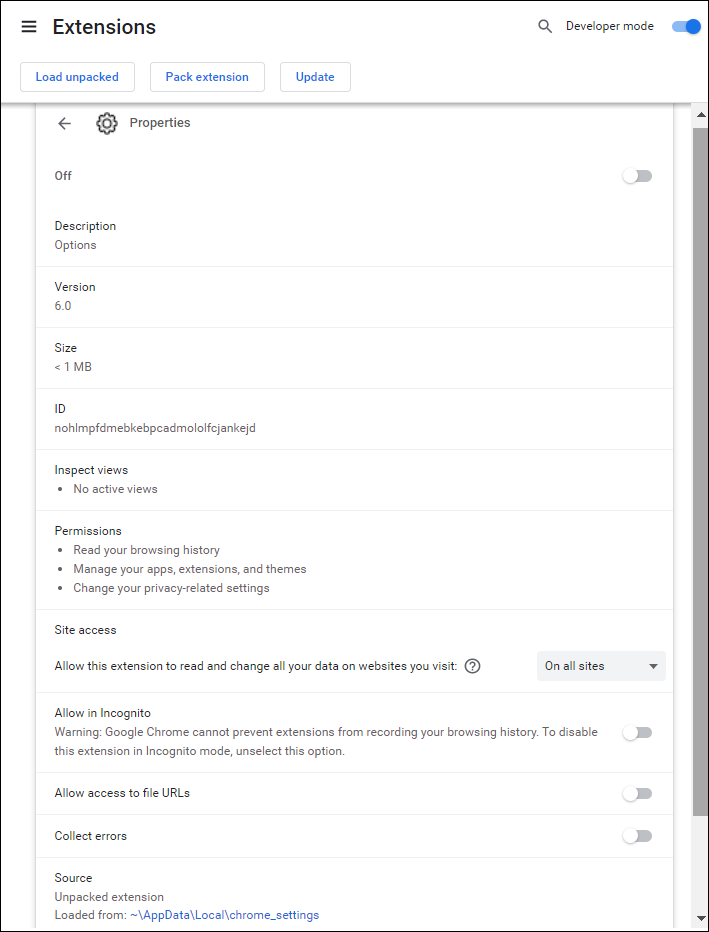This image is a screenshot of a computer screen displaying the "Extensions" page in a web browser. At the top of the page, the "Developer mode" option is clearly visible, highlighted in blue to indicate that it is turned on. Below this, there are buttons labeled "Load unpacked," "Pack extension," and "Update," each situated within its own rectangular section with a blue outline.

Further down, there is a "Properties" section, identifiable by a gear icon on a white background. Beside this icon, the toggle switch is set to the "off" position, which is confirmed by the slider being moved to the far right. 

Continuing down, there is an area labeled "Description" with an "Options" link underneath it. This section also includes details such as "Version: 6.0" and "Size: Less than 1 MB." There is an "ID" section that contains a long string of lowercase letters and numbers, followed by a "Inspect views" area which states "No active views."

Further down the page, a "Permissions" section lists the following capabilities granted to the extension: "Read your browsing history," "Manage your apps, extensions, and themes," and "Change your privacy-related settings." 

Finally, a "Site access" section indicates that the extension has permission to "Read and change all your data on websites you visit," with the setting applied to "On all sites." The page continues with additional details and options below.